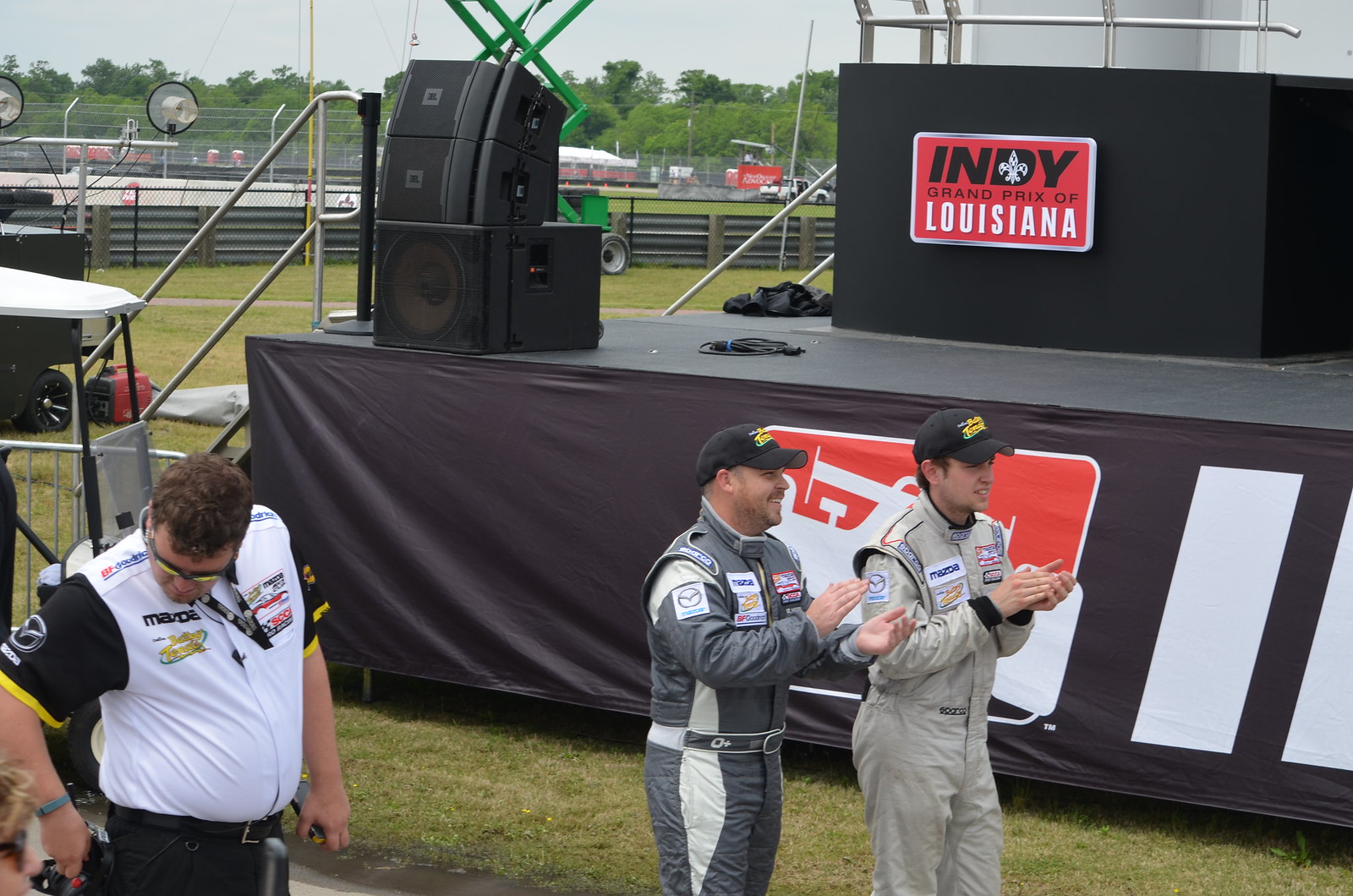In this full-color photograph of an outdoor event, three Caucasian men—presumably professional race car drivers—stand in the foreground. The scene is set against the backdrop of a racetrack, marked by tall fencing, stadium-like seating, and a variety of metal rods. Two of the men are dressed in racing jumpsuits adorned with advertising badges; one wears a silvery-gray suit, while the other dons a darker gray suit with white detailing. Both have billed hats. The third individual, positioned to the far left, sports a white jersey decorated with various logos, paired with work pants and a belt. He also has a watch on his left wrist. The men stand in front of a stage with speakers and a black podium that reads "Indy Grand Prix of Louisiana." In the background, a close-cropped field, which suggests late summer, is visible along with green shrubbery, lights, and more structural details of the racetrack. Two of the men appear to be clapping and are looking off to the right. It is clearly daytime.